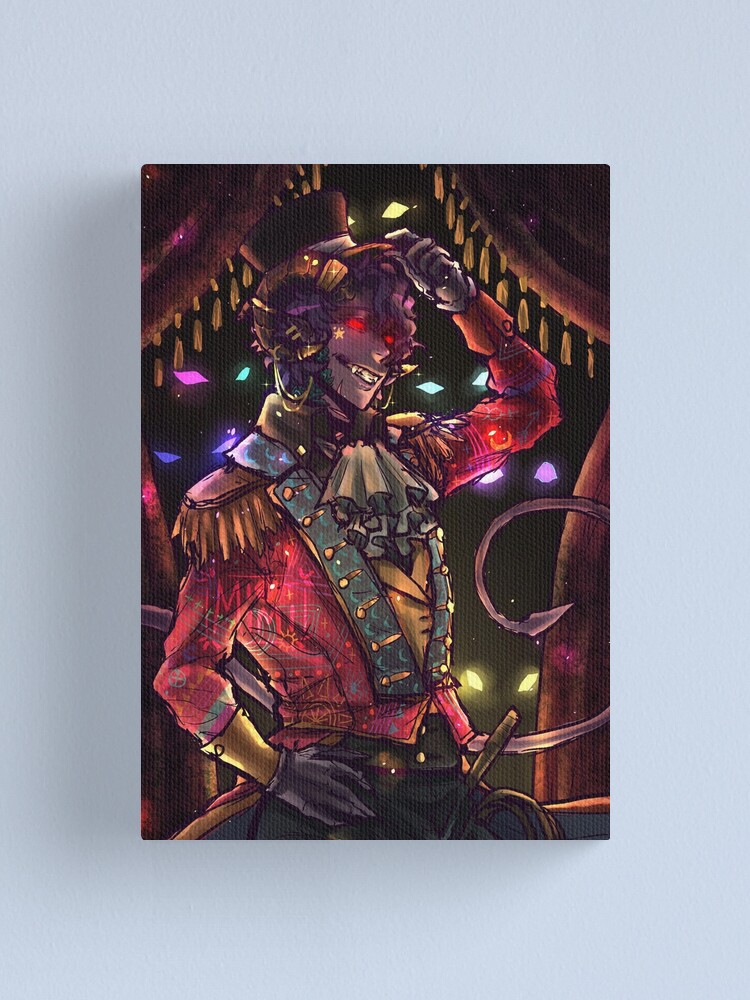The photograph, rectangular with its longer sides oriented vertically, showcases a large painting hung against a light blue, textured wall. The painting itself, also rectangular in shape but elongated similarly, features a striking depiction of a humanoid demon creature set against a dark, mysterious backdrop. Visible from the waist up, the demon commands attention with glowing red eyes, purple skin, and large ram-like horns curling around its pointed ears. Clad in traditional ringmaster attire, the creature dons a red long sleeve shirt adorned with gold-tasseled shoulder pads, blue sections flanking a gold-buttoned central strip, and a white ruffled ascot. A matching top hat perched between its horns completes the sinister ensemble. Additionally, the creature brandishes pointed fangs and a mischievous smile. Its long, purple tail, ending in a triangular point, coils dynamically around the figure, enhancing the artwork's eerie yet captivating aura. Although evocative of anime and fantasy genres, the painting retains a unique, personalized style, suggesting it could be part of a collection available through custom poster vendors.